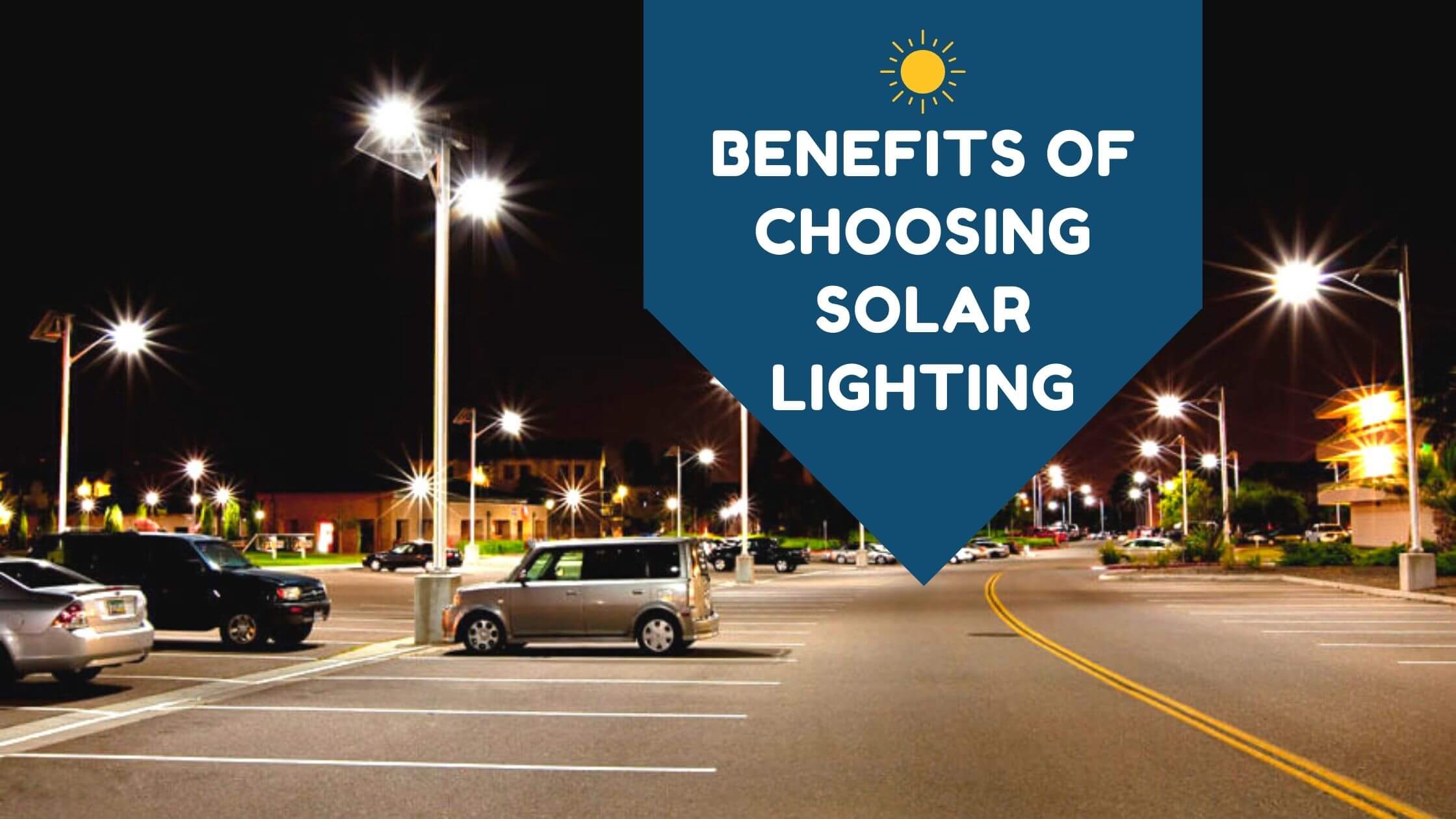This image depicts a suburban parking lot under the cloak of night, casting an almost desolate and eerie atmosphere. The parking lot, paved in dark grey asphalt, holds only a few cars scattered under the bright streetlights. These streetlights, exaggerated through heavy Photoshop effects, gleam intensely, resembling stars against the stark night. A road, devoid of life, runs along the right side of the image, emphasizing the isolation of the scene.

In the background, silhouettes of a few indistinct buildings and trees can be seen, slightly warming the otherwise cold and empty ambiance. Dominating the top of the image, a bold blue banner with a shape reminiscent of an upside-down house contains the white, uppercase text: "BENEFITS OF CHOOSING SOLAR LIGHTING." Adding a touch of whimsy, a small, cartoonish yellow sun sits atop the letter 'F' in 'BENEFITS', further drawing attention to the message.

The ad combines detailed visual elements with a clear, compelling title, effectively promoting the advantages of solar lighting through an artistic and somewhat surreal nighttime setting.